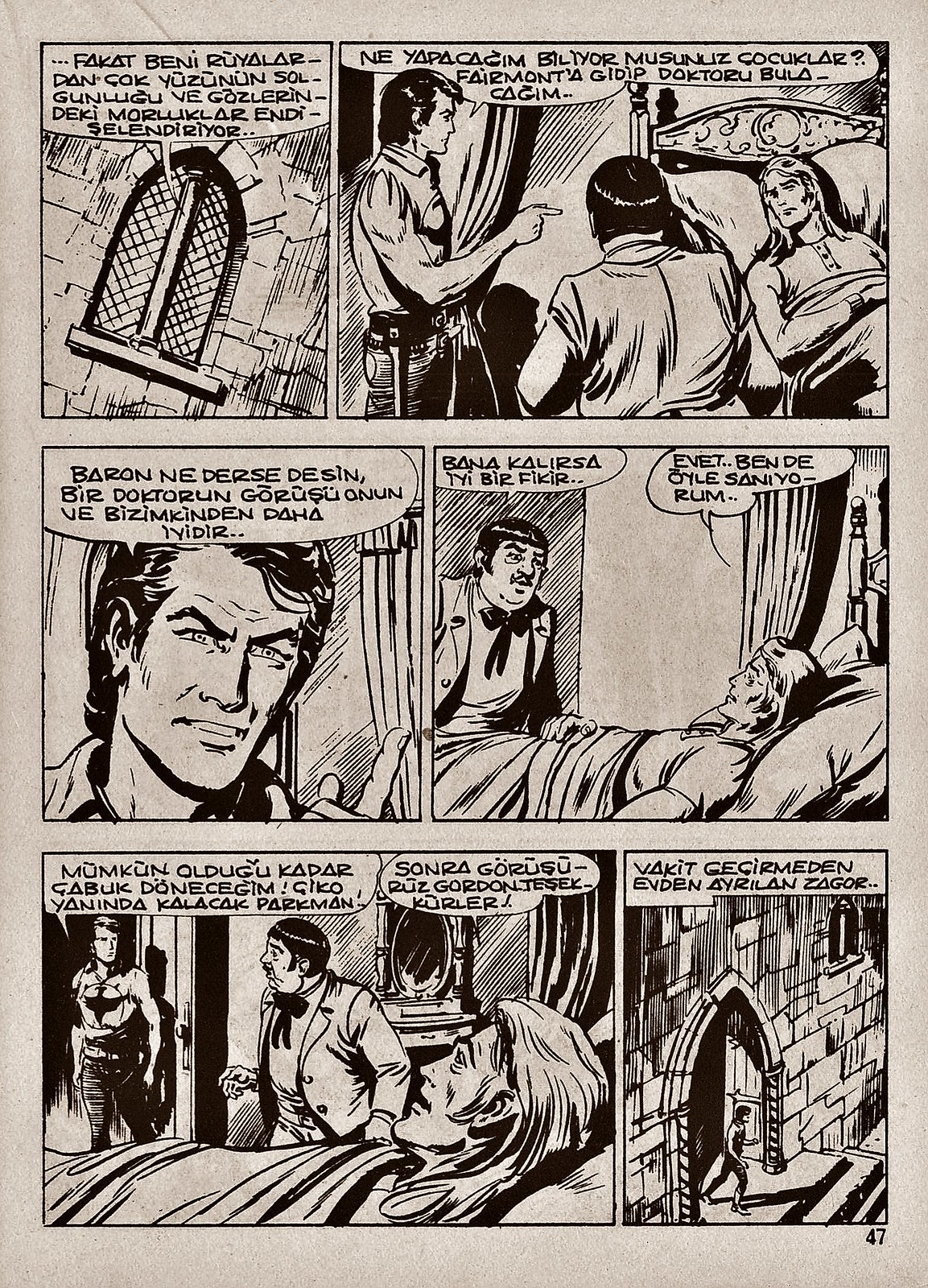This black-and-white comic strip is a single page, specifically page 47, and is written in Turkish. It is laid out in three rows of panels, with each row containing two panels. The first panel features an old, rounded-top castle window. In the second panel, two men—one young and muscular, the other older, short, and round with a peculiar square bowl haircut—stand beside a bed with a person lying in it who appears to be young and muscular. The third panel offers a close-up of the young, muscular man's face. In the fourth panel, the older, stout man is shown talking to the person in the bed, who may be either young or an older individual who was formerly muscular. The fifth panel illustrates one of the standing men positioned at a doorway, seemingly about to exit the room. The final panel captures this man leaving through a castle door. The narrative suggests that the person in the bed might be of noble or royal status, though their exact situation is unclear. The overall atmosphere of the comic suggests a medieval or fantasy setting.